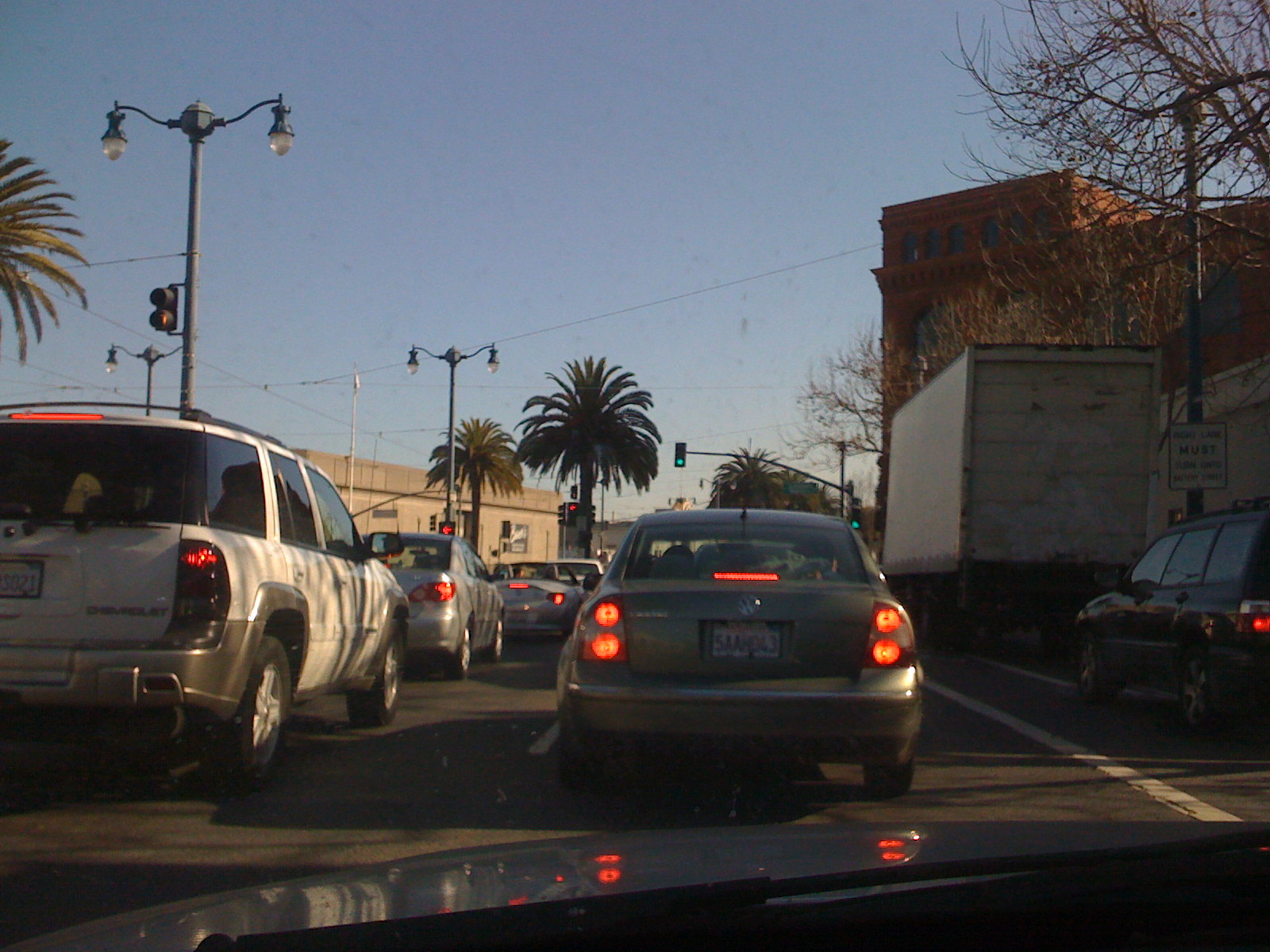This is a daytime photo taken from the front seat of a car in a traffic queue, captured in an American city. The bonnet of the car is visible at the bottom, and we are positioned in the middle lane of a three-lane road. Directly in front of us is a Volkswagen Passat with its brake lights on. To our right, there is a Subaru Forester and a large lorry ahead of it, while in the left lane, there is a Chevrolet SUV and a gray sedan in front of it, followed by a white convertible.

The traffic lights in the distance are green for the middle lane and the lane to our right, but red for the left lane, suggesting that the cars are about to start moving. The sky is a hazy light blue, creating a soft backdrop for the scene. Several palm trees are noticeable, one encroaching from the left edge of the image, and a couple more near the traffic lights. The street lighting consists of old-fashioned lamps with large poles and long arms extending outwards.

On the right side of the image, beyond the lorry, stands an orange-brick building with several clear-glass windows. In the further distance, a beige, single-story warehouse-like structure is visible. The overall atmosphere is that of a typical urban environment, underlined by the mix of everyday vehicles and the anticipation of the traffic signal changing.